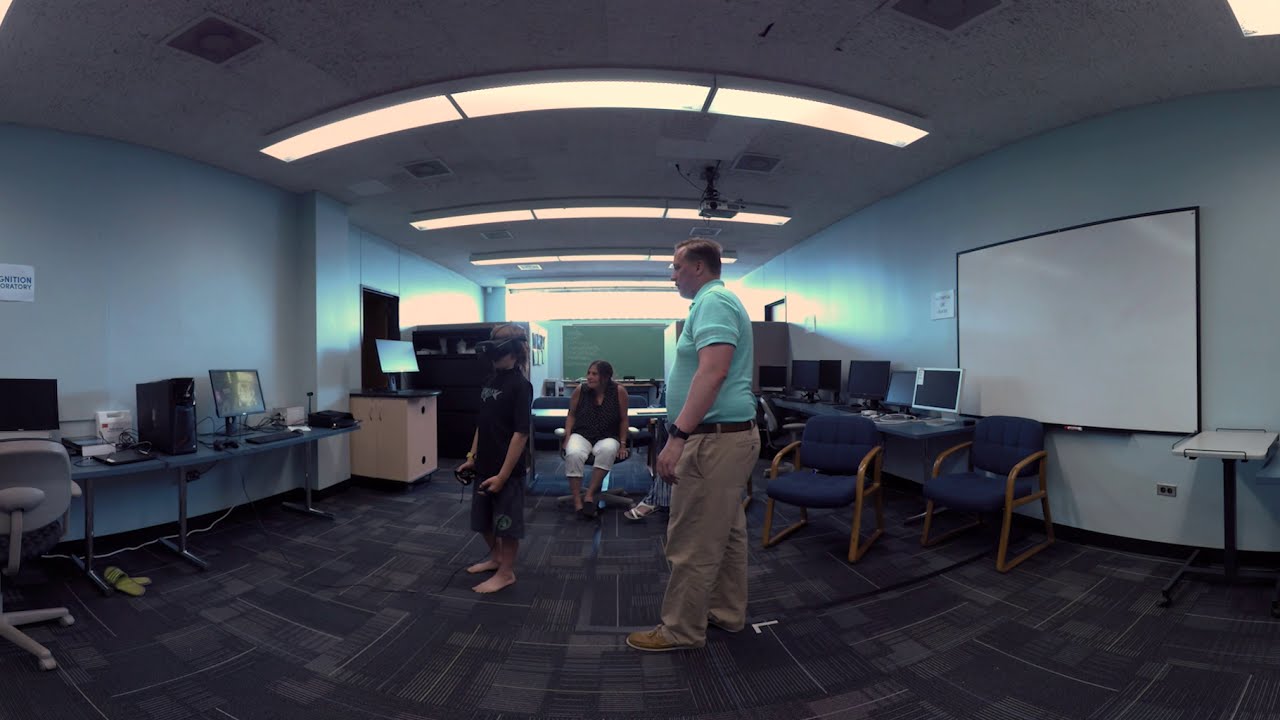In a spacious computer lab classroom, three people are the focal point of the image. On the left side stands a young boy, around 12 years old, who has short brown hair and is wearing a black short-sleeved shirt and green shorts. He is barefoot and equipped with a black VR headset and holding controllers in both hands. The boy is facing towards the left side of the image. In the center, there is a woman with dark brown hair, seated on a small blue chair. She is dressed in a black sleeveless top, white capri pants, and black sandals, observing her surroundings, possibly a monitor. To the right and closer to the foreground, stands a slightly heavier-set man, appearing to be in his 40s. He has short brown hair and is dressed in a light green polo shirt, khaki pants, and brown shoes, with a black watch around his wrist. This man, who could potentially be the boy's father, has his body turned to the left, attentively watching the boy. Surrounding them are numerous computer stations; on the left wall, there is a long blue table with several computers and gray desk chairs. On the right side, a similar setup is mirrored with blue chairs featuring brown trim. A whiteboard is mounted on the right wall, and the room is illuminated by multiple rows of long, fluorescent lights across the ceiling. An additional detail is the presence of what seems to be another person, with only a foot visible in the frame, hinting at more activity within the room.